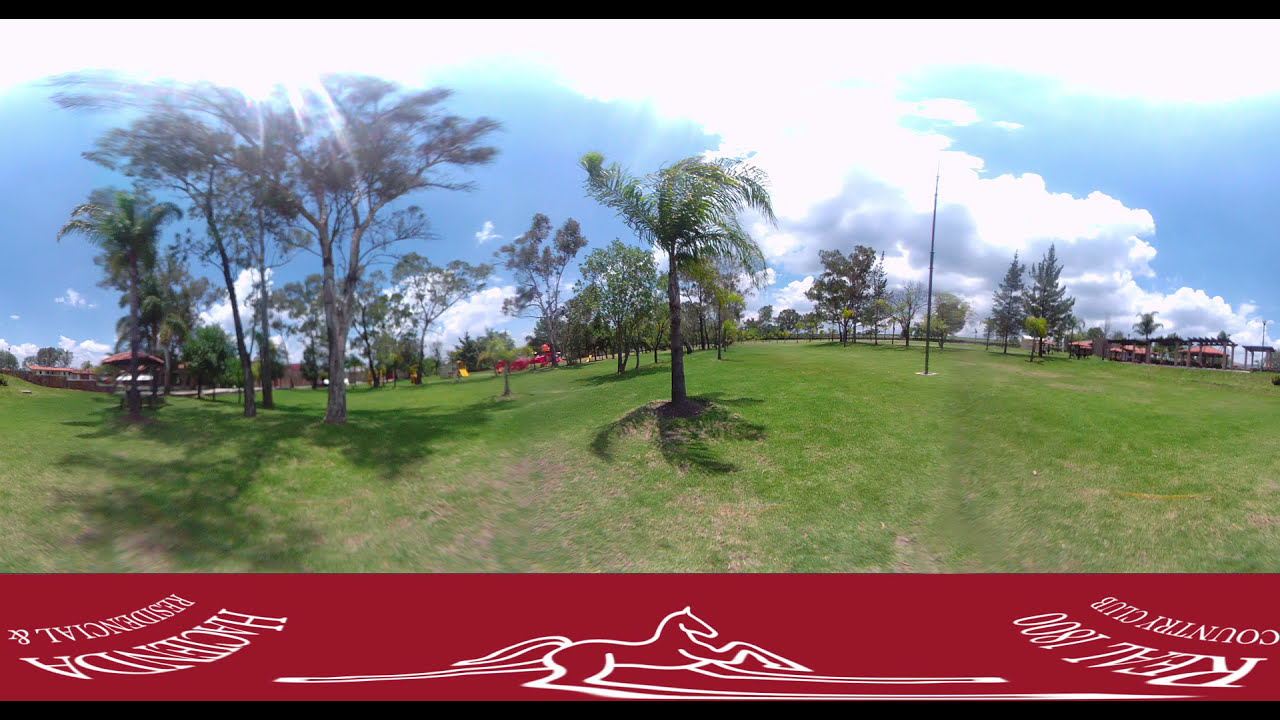This photograph captures a wide-angle view of a well-kept lawn expanse, possibly a golf course or park, adorned with a mix of palm trees and regular trees casting visible shadows in the bright, sunny daylight. The lawn, while mostly green, exhibits patches of brown grass. A notable element is a pole sticking vertically out of the ground, potentially marking a golf hole. The backdrop features several brick buildings located on both the left and right sides in the distance, accompanied by some structures that resemble outdoor picnic shelters or perhaps playground equipment. The sky is predominantly blue with a combination of light gray, darker gray, and white puffy clouds dispersed across it. At the bottom of the image, there is a red banner with white text reading "Real 1800 Country Club" and "Hacienda Residential," along with a drawing of a white horse, though the text appears distorted.